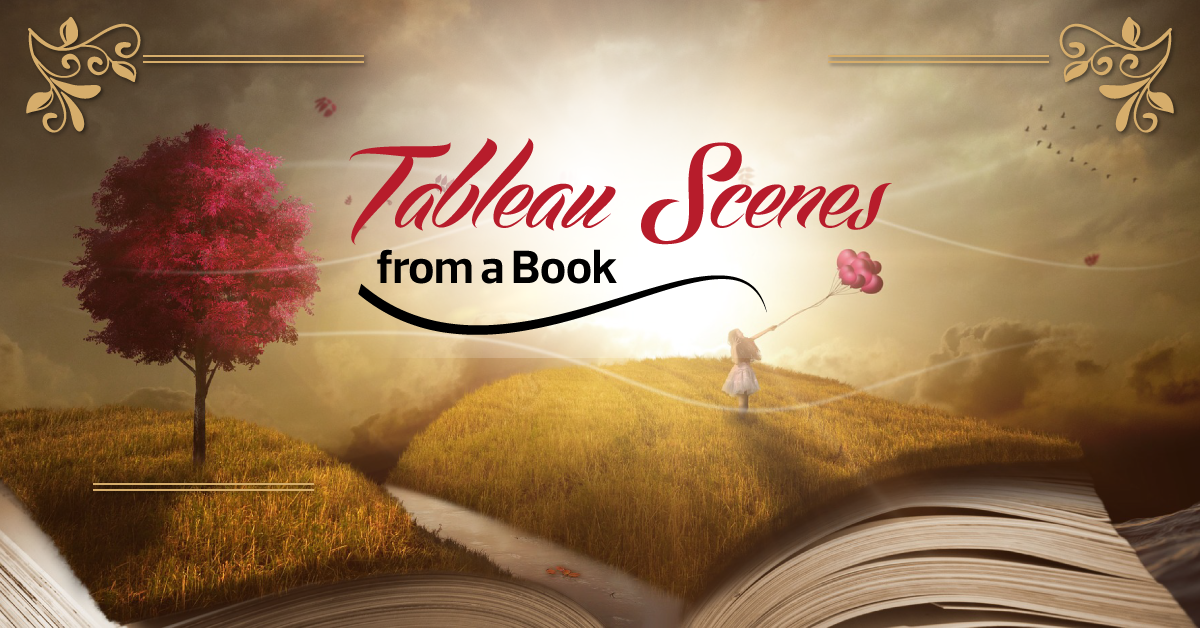The image appears to be a detailed and imaginative book cover, designed in a collage or illustration style reminiscent of Photoshop artwork. At the top, bold red text reads, "Tableau Scenes," followed by a subtitle in black, "From a Book," which is underlined by a curved black line. The upper corners feature intricate golden vines, with leaf-like designs that resemble stamps.

The main scene depicted on the cover blends literary elements with a dreamlike nature setting. An open book serves as the foundation, with the right and left pages transforming into a hilly field of multicolored grass, ranging from brown to green. On the left side of this field, there is a small tree with vibrant, dark pink leaves.

On the far right, a young girl in a white dress holds a bunch of pink balloons tied with strings. She stands facing away from the viewer, her figure small but capturing attention as she walks through the field. In the background, the sky is filled with dark gray clouds, though a bright white and yellowish light, resembling the sun, pierces through the center. Birds can be seen flying across the sky above the girl.

The artwork creates an ethereal and whimsical scene, where the open book seamlessly melds with nature, symbolizing a journey that starts from the pages and transcends into an imaginative world.